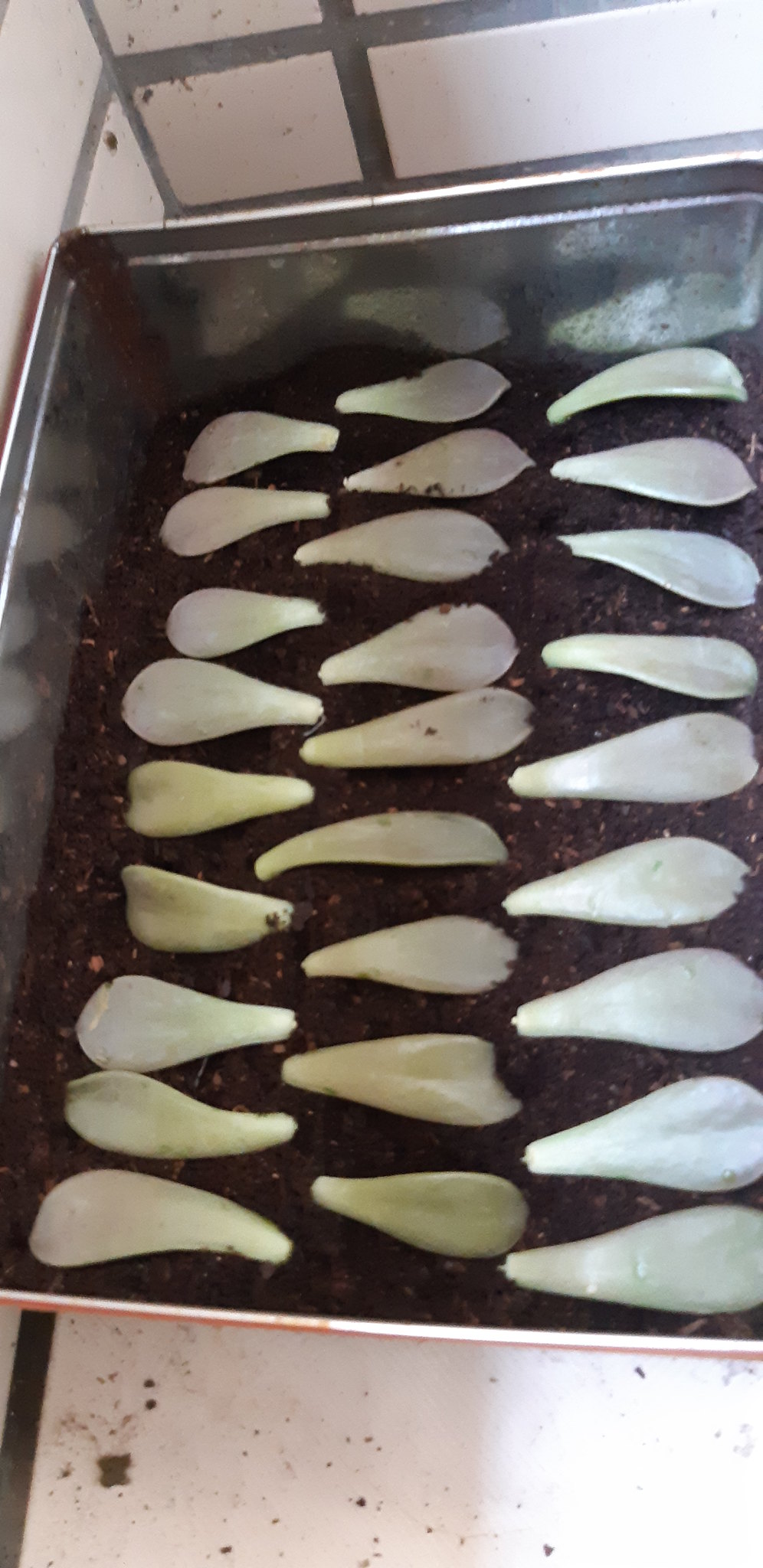The image depicts a large rectangular metal container situated on a somewhat dirty white table. Inside this container, there are three neatly spaced columns of small, white, pearl-like objects, each column containing approximately six to ten items. These objects are triangular-shaped and appear to be embedded in a dark, dirt-like substance. The metal container reflects these objects, adding to their prominence. Behind the container, a white wall with gray rectangular dividers serves as the background.